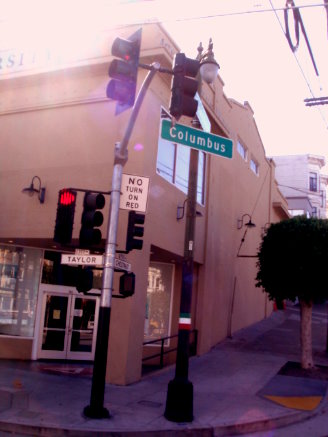This real-life image captures the intersection of two streets, focusing primarily on the sidewalk in front of a beige khaki-colored building at the corner. The left of the frame features a traffic light post with multiple traffic lights facing different directions. One of the traffic lights, facing the camera, is illuminated red. Attached to this post is a sign that reads "No Turn on Red" in black letters on a white background with a black border. Below the traffic light, a street sign with "Taylor" written in black letters on a white background is visible. 

On the right side of the image, a lamp post stands, equipped with a streetlight. Attached to this lamp post is a green street sign with "Columbus" inscribed in white letters, also featuring a white border. The building at the corner showcases a reflective double-door entryway, making it difficult to see inside. Small hanging lamps adorn the building's façade. To the right, a tree is planted in a rectangular dirt cutout on the sidewalk. The edge of the sidewalk and a small section of the street are visible towards the bottom right of the image.